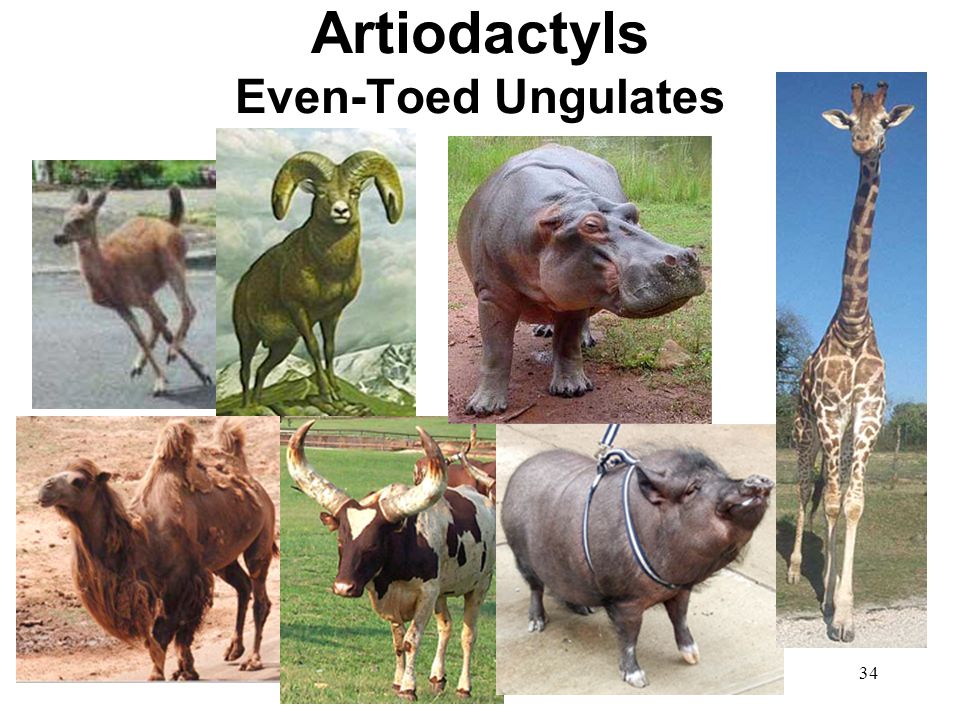The image features several photographs of animals arranged on a white background with black text. At the top, centered, are the words "Arteodactyls" followed by "Even-toed Ungulates," both capitalized. Below the text, there are seven animal photographs arranged in a specific layout. On the left three-quarters of the image, there are two rows of three pictures each. The top row includes a deer on the left, a painting of a bighorn sheep in the center, and a photograph of a hippopotamus on the right. The bottom row features a two-humped camel on the left, a large cow with long horns in the center, and a pot-bellied pig on the right. On the right side of the image, occupying the space of two of the left-side pictures, is a tall rectangular photograph of a giraffe. Below the giraffe, in small black text, is the number 34.